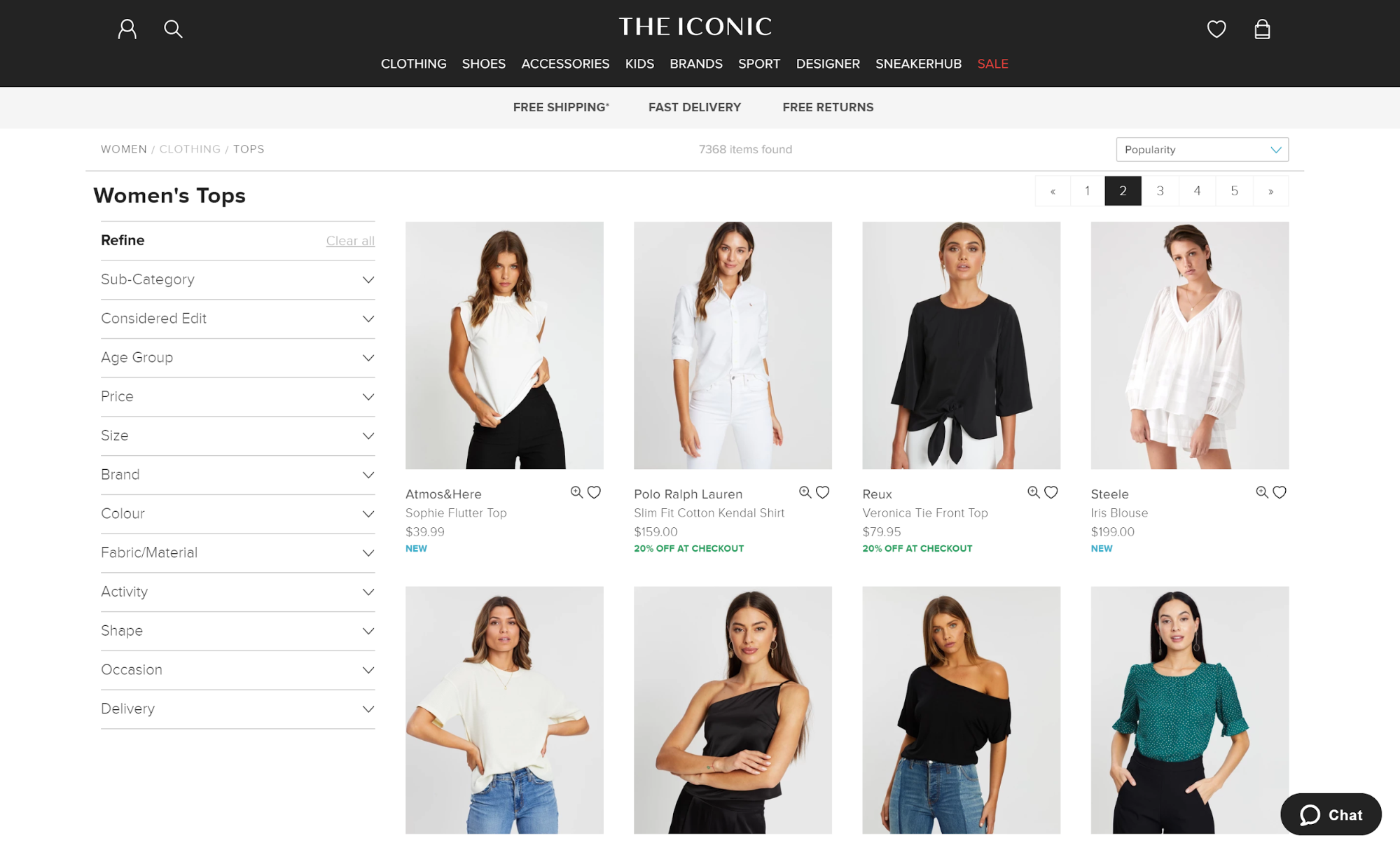Screenshot of The Iconic Fashion Sales Website: The image showcases the homepage of The Iconic, a popular fashion sales website. The top of the screen is dominated by a dark gray banner with "The Iconic" prominently displayed in the center. This banner also features various shopping categories: Clothing, Shoes, Accessories, Kids, Brands, Sport, Designer, Sneaker Hub, and Sale, with the word "Sale" highlighted in red for emphasis. Below the banner, central text advertises customer benefits: "Free Shipping, Fast Delivery, and Free Returns."

The main content area displays two horizontal rows with four thumbnails each, showcasing a variety of women modeling different shirts. Each woman features a unique style of top, with most having dark or almost black hair and light skin. Specifically, four women are dressed in white shirts, three in black shirts, and one in a green shirt.

On the left side of the screen, a vertical menu allows users to refine their search for women's tops. The options include refining the search or clearing all filters, and allows further narrowing down by subcategory, considerations, edits, age group, price, size, brand, color, fabric/material, activity, shape, occasion, and delivery options.